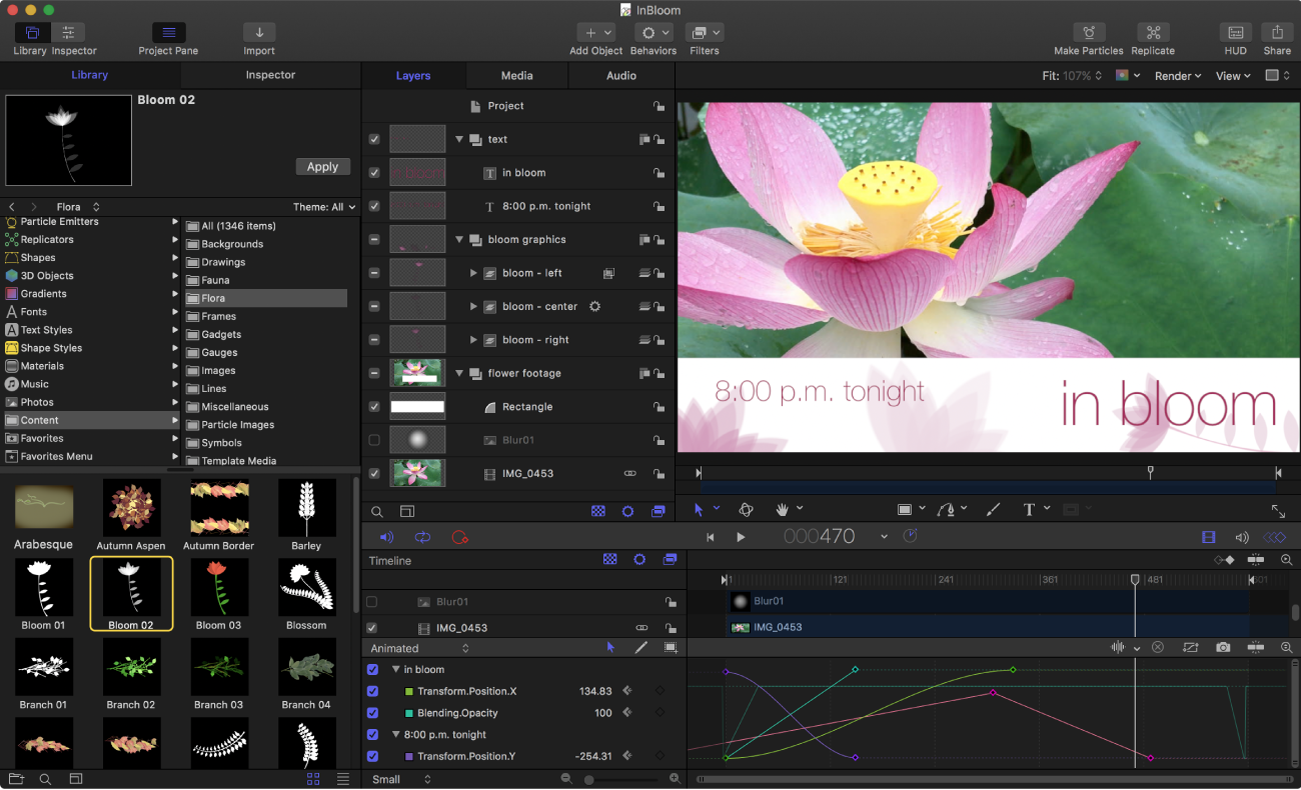The image is a detailed screenshot from a computer screen—likely an Apple computer—showing an advanced photo or video editing software such as Adobe After Effects or Photoshop. The screen is filled with detailed information, including numerous menus and taskbars, with approximately 50 different tabs that allow the user to modify graphics, images, color ranges, orientations, and import projects. 

Taking up about the right-hand quarter of the screen is a prominent and detailed image of a large water lily, with petals in shades of pinkish-purple and white, and a vibrant yellow stamen at the center. Behind the flower are green leaves, adding depth to the image. The photograph includes a caption that reads "8 PM tonight in bloom," which appears on a white border at the bottom of the image.

Adjacent to the image, the screenshot shows various audiographs and media layers related to the project, indicating ongoing editing processes such as color saturation and color mixing adjustments. The user interface is predominantly displayed in black and white text, reinforcing the professional nature of the software in use. The file name noted in one of the tabs is "Balloon02," and the entire setup indicates a highly customizable and intricate editing environment designed for detailed image or video work.